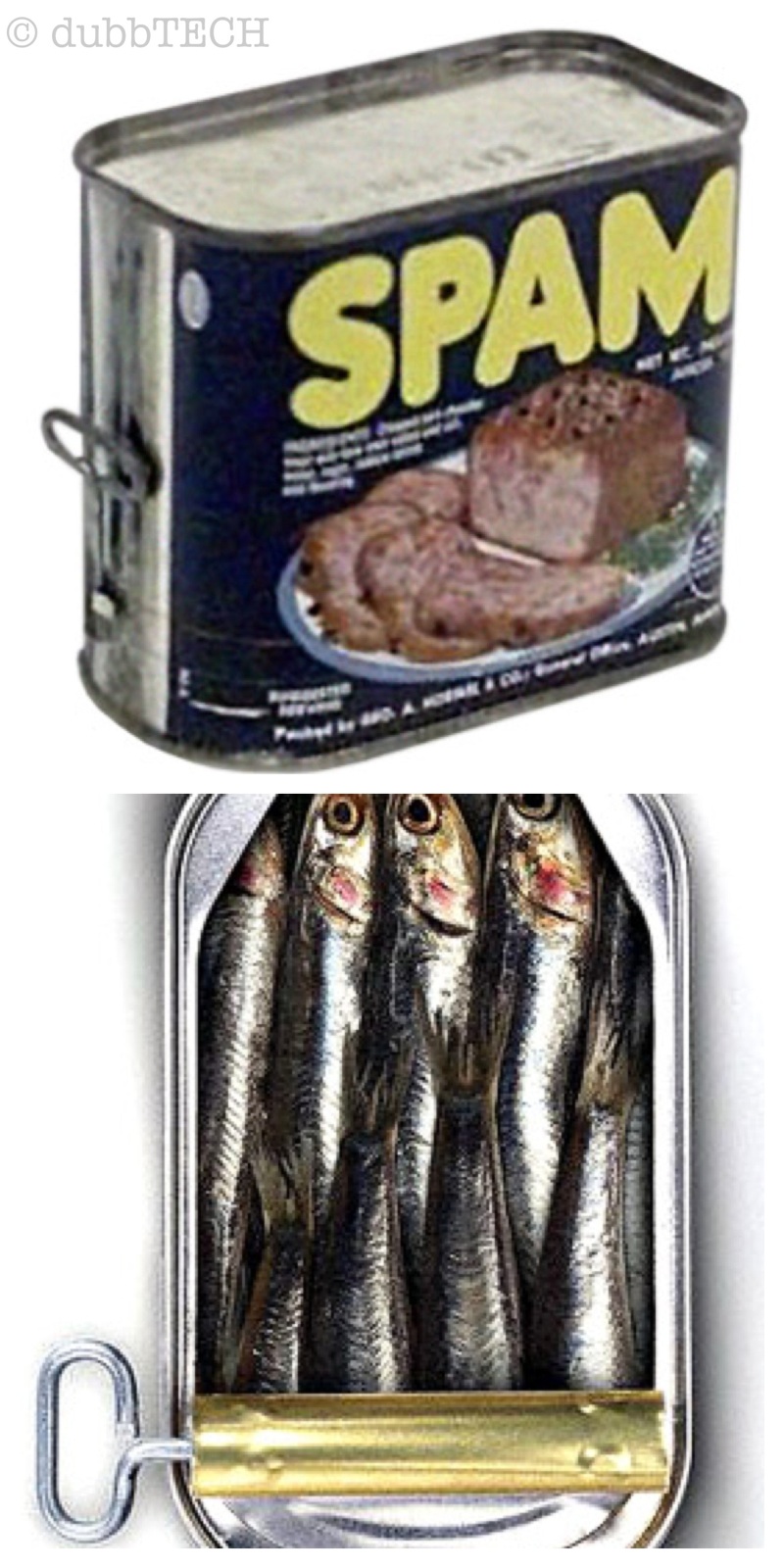The image is a composite of two distinct photos, one above the other, both in portrait orientation. The top half features a slightly tilted, unopened can of Spam with the classic blue label and yellow "Spam" text. The front of the can depicts a loaf of Spam with four slices cut and arranged on a plate. Attached to the left-hand vertical side of the can is a small key intended for opening it. Positioned on a white background to the left of the top of the Spam can, there is a silver, circular copyright symbol followed by the text "Dub" in lowercase and "TECH" in uppercase.

The bottom half of the image shows an opened can of sardines from a top-down perspective. The lid of the sardine can has been rolled back using the built-in key, revealing sardines neatly packed inside. The visible sardines are arranged in rows, with tails at the bottom and heads at the top, each with a visible eye. The overall image juxtaposes these two food items, highlighting their packaging and the method used to open them.